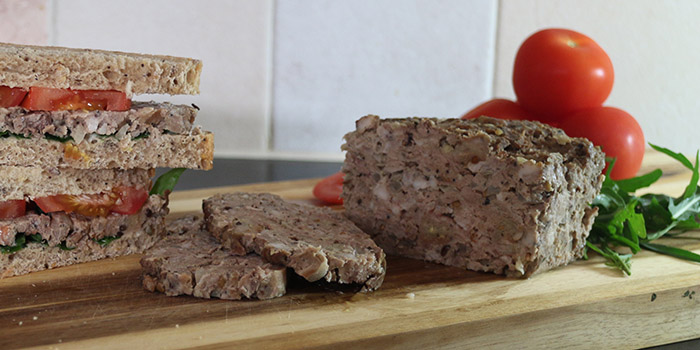This color photograph showcases a rustic presentation of sandwiches and meatloaf on a wooden board set beneath a wooden shelf. On the left side of the board, several sandwiches are stacked, each featuring layers of assorted meats, fresh tomatoes, and dark brown bread. Positioned centrally, two slices of dark bread are neatly arranged, suggesting possible meatloaf between them. To the right, a larger, uncut chunk of meatloaf is partially sliced at the edge, exposing its interior. Just beyond the meatloaf, a small pile of tomatoes is visible, with three whole ones stacked and another partially sliced piece peeking out from behind the meatloaf on the left. Complementing this arrangement, a touch of greenery adds a fresh accent beneath the tomatoes. The background consists of light grey tiles at the top, transitioning to darker tiles at the level of the wooden board. A small triangle of black is noticeable in the lower right-hand corner of the image, adding contrast to the overall composition.